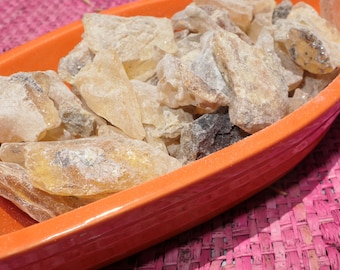In this close-up photograph, an oblong, tangerine-colored ceramic vessel, reminiscent of a canoe, is prominently displayed atop a woven pink wicker or rattan mat. The vessel is filled with a disordered collection of rough, unprocessed crystals and rocks, ranging in size from about half an inch to three inches long. The crystals exhibit a variety of hues, including off-white, yellow, and gray, with some appearing fairly clear while others exhibit darker tones. Among the assortment, there's one particularly notable rock that appears almost entirely gray, and one with markings that resemble a line-drawn face, adding a whimsical touch to the scene.